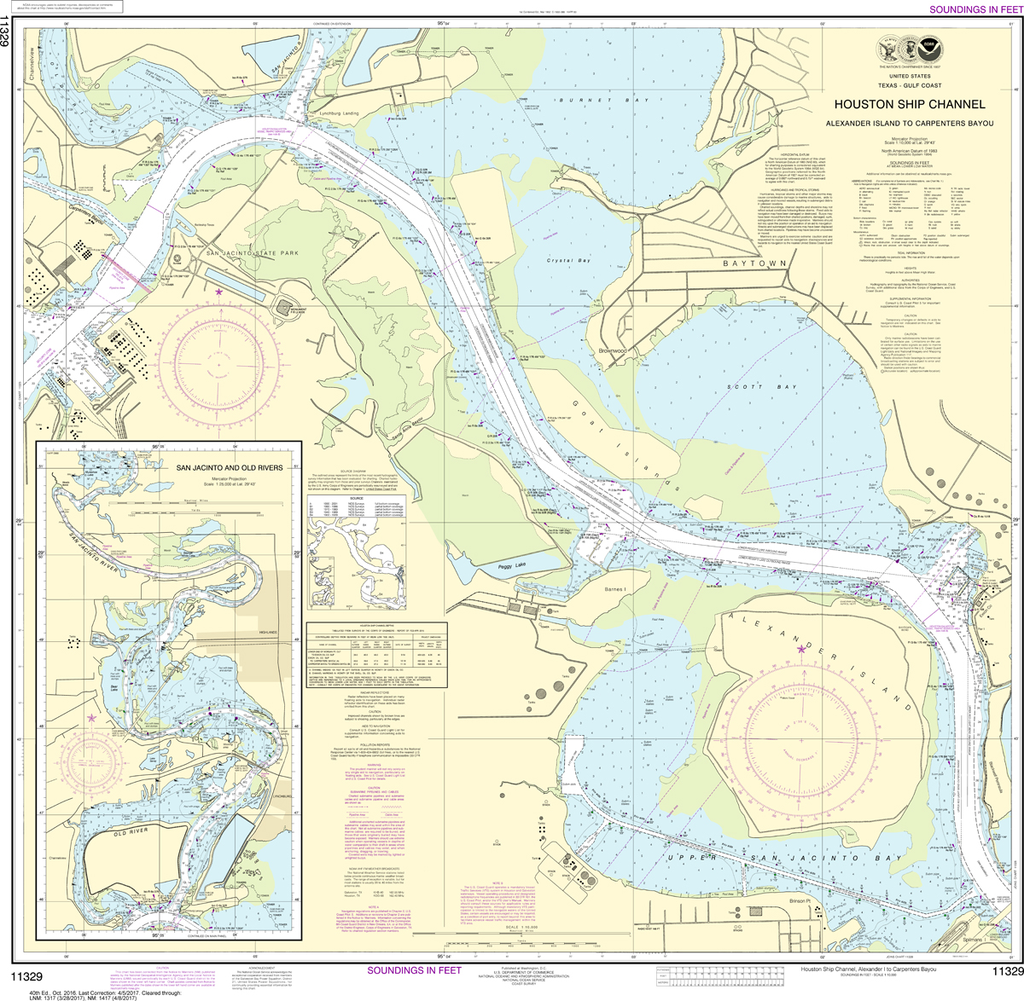This is a highly detailed, faintly rendered map of the Houston Ship Channel, spanning from Alexander Island to Carpenter's Bayou. The main channel is prominently marked in white, flanked by light blue water areas and various land masses depicted in shades of beige, yellow, and light green. Notable features include a bridge cutting through the center and multiple lines and compasses for navigation. The top right corner prominently displays "Houston Ship Channel" with an additional note, "Soundings in Feet," at the very top. The lower left corner contains a zoomed-in, more detailed section of the map, including several keys and annotations, aiding in the identification of features that are too small to read on the main map. This artistic representation, which could be a sketch or a photograph with a muted look, provides a comprehensive view of the area with intricate details throughout.